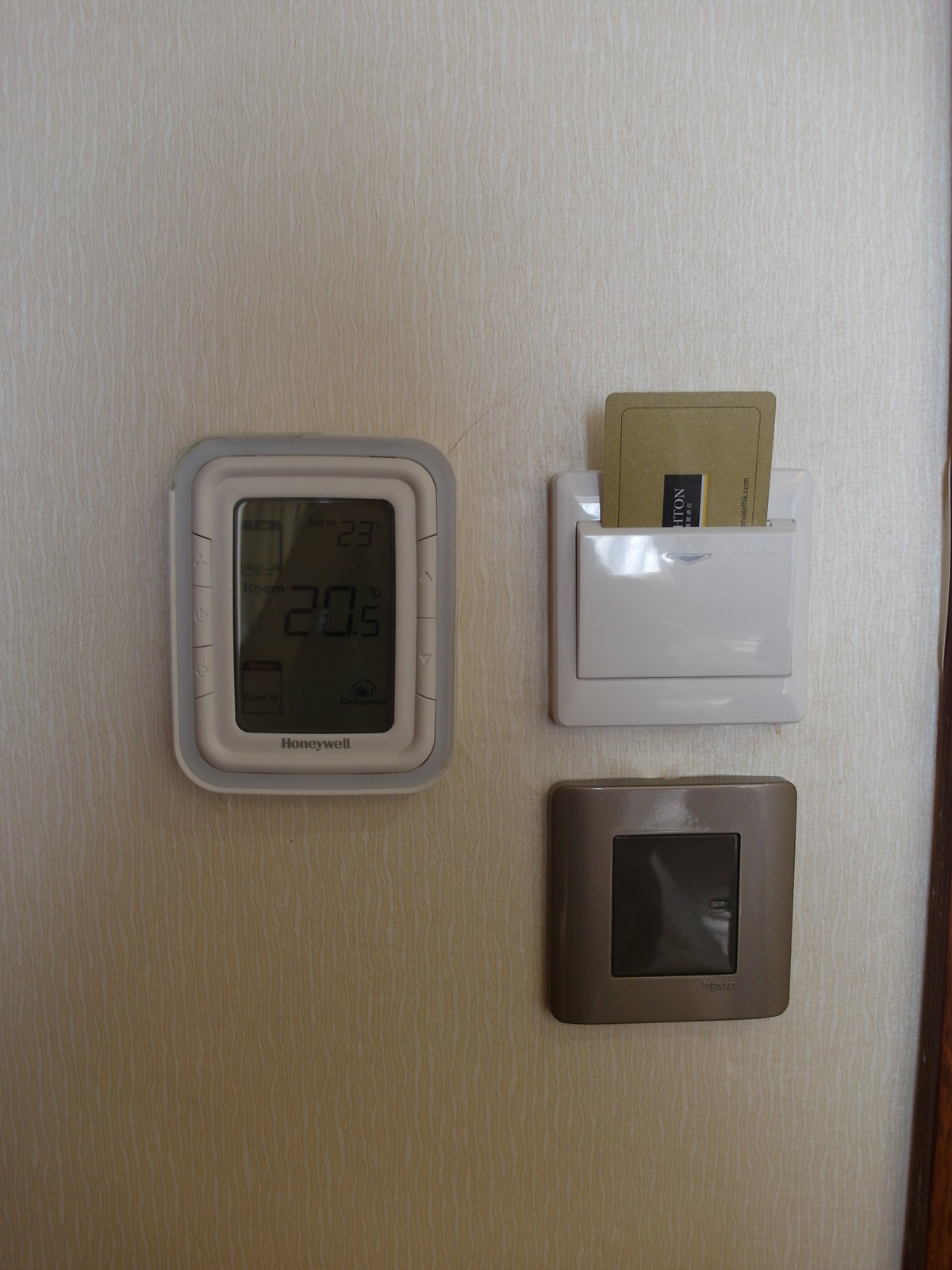This photograph captures three distinct objects mounted on a pristine white wall, displaying subtle but noticeable shadowing and gently wavy lines descending its surface. On the left, a Honeywell digital thermostat is affixed to a grayish-white faceplate. The thermostat itself comprises a white body and a digital screen, which prominently features black numbers and text, suggesting current settings or readings.

To the right, two additional objects are mounted vertically, one above the other. The upper object is a white, glossy device with a sleek design, supporting a golden and black card resting in its built-in pocket. Beneath this, a darker silver, square-shaped object resides, with a central screen of a muted gray hue that currently displays no active images or text. Each object reflects ambient light, adding a subtle gleam to the scene.

In the margin of the photo, a narrow slice of a wooden door frame is visible, enriched with shadowing that adds depth and dimension to the overall composition.